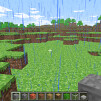Here is the revised and detailed description based on the provided information:

---

Screenshot from the game Minecraft: The player is depicted carrying a block of cobblestone while navigating a grassy terrain. Their inventory bar at the bottom of the screen is filled with various building materials, including different types of stone and wood, as well as an apple. The landscape features a slight hill directly in front of the player, but the rest of the area is mostly flat. It appears to be raining, with visible water droplets both near and far. Despite the rainy weather, the sky remains relatively light blue, filled with clouds. In the distance, trees dot the horizon, adding to the natural scenery. There are no visible enemies in the scene. The cursor, a white plus sign, is centered on the screen. An indistinct figure, possibly an animal, is faintly visible in the back right corner of the image, though the small size of the screenshot makes it difficult to identify.

---

This caption provides a clearer and more structured description of the Minecraft screenshot.